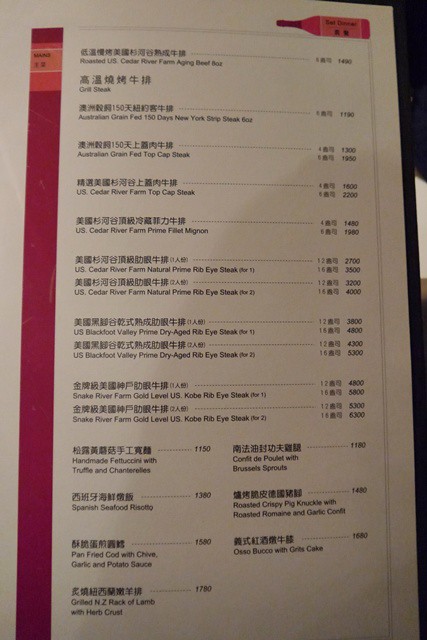This photograph captures a neatly arranged restaurant menu designed as a vertical, elongated rectangle predominantly in white with black text. The top right corner of the menu features an image of a wine bottle, tilted on its side with the bottle's neck pointing left and the base to the right. The bottle is a vivid red color and is adorned with text that appears to be in Chinese. Complementing this, a matching red strip runs down the left side of the menu, adding a cohesive splash of color.

The menu is clearly organized, with the top section dedicated to main dishes, prominently featuring steak options. Each item is listed first in Chinese, followed by its English translation and corresponding prices to the right. 

The bottom portion of the menu showcases an array of seven alternative choices, offering diners a varied selection beyond steak. Similar to the main dishes, these items are presented with their names in Chinese and English. The well-structured layout and bilingual presentation cater to a diverse clientele, enhancing the menu's accessibility and appeal.